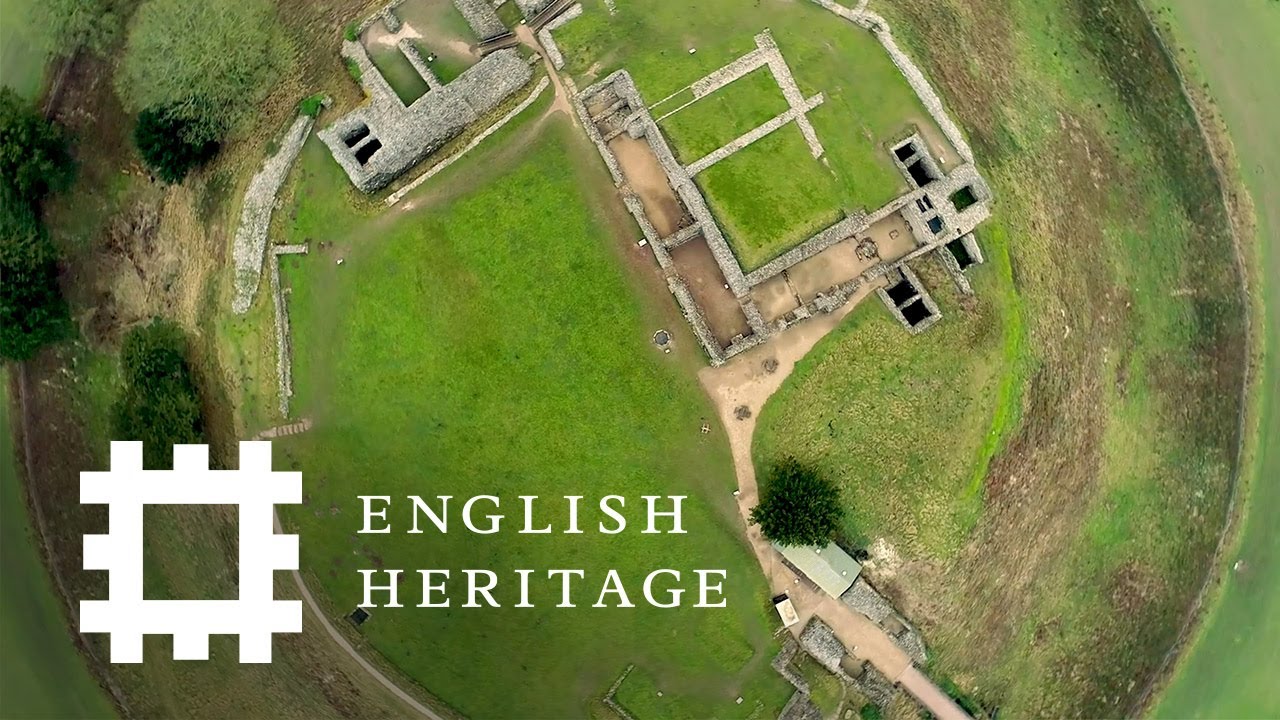This aerial overhead photograph captures the intricate details of an ancient stone fortification, likely an old castle or historical site, resting amidst lush green grass. The remnants of the stone walls create a labyrinthine pattern with right angles and numerous smaller rooms, revealing centuries of architectural evolution. Dark green patches and dirt trails crisscross the structure, exposing pathways and worn areas of the hill it occupies. A modern structure with a light green roof is located towards the bottom of the image, contrasting with the ancient stones. The entire scene is enclosed in a circular area, with the circle extending beyond the image's boundaries at the top and bottom. The tops of green trees frame parts of the circle, adding natural elements to the man-made relics. Superimposed on the bottom left of the image is a white square logo with crenellations, accompanied by the text "ENGLISH HERITAGE" in all capitals, signifying the site’s historical and cultural importance. This image, likely taken from a drone or helicopter during daylight, provides a detailed and immersive view into the preserved and excavated elements of this ancient heritage site.